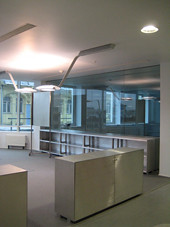The small thumbnail image depicts an empty, dimly lit office or library space with white walls and a gray floor. Central to the scene is a partition that obscures some empty bookshelves, showing us the back side of one, which has sections appearing like cardboard. To the right, there’s a reflection from what seems to be a glass or mirrored wall. Light fixtures, including a circular one on the right wall and another hanging from the middle of the ceiling, illuminate the room. The image also reveals a street scene with other buildings through the windows. The area feels deserted, with no people, tables, or chairs in sight, just an ambiguous object, possibly a cart or heater, against a far wall, and an adjacent dark room that mirrors the emptiness.